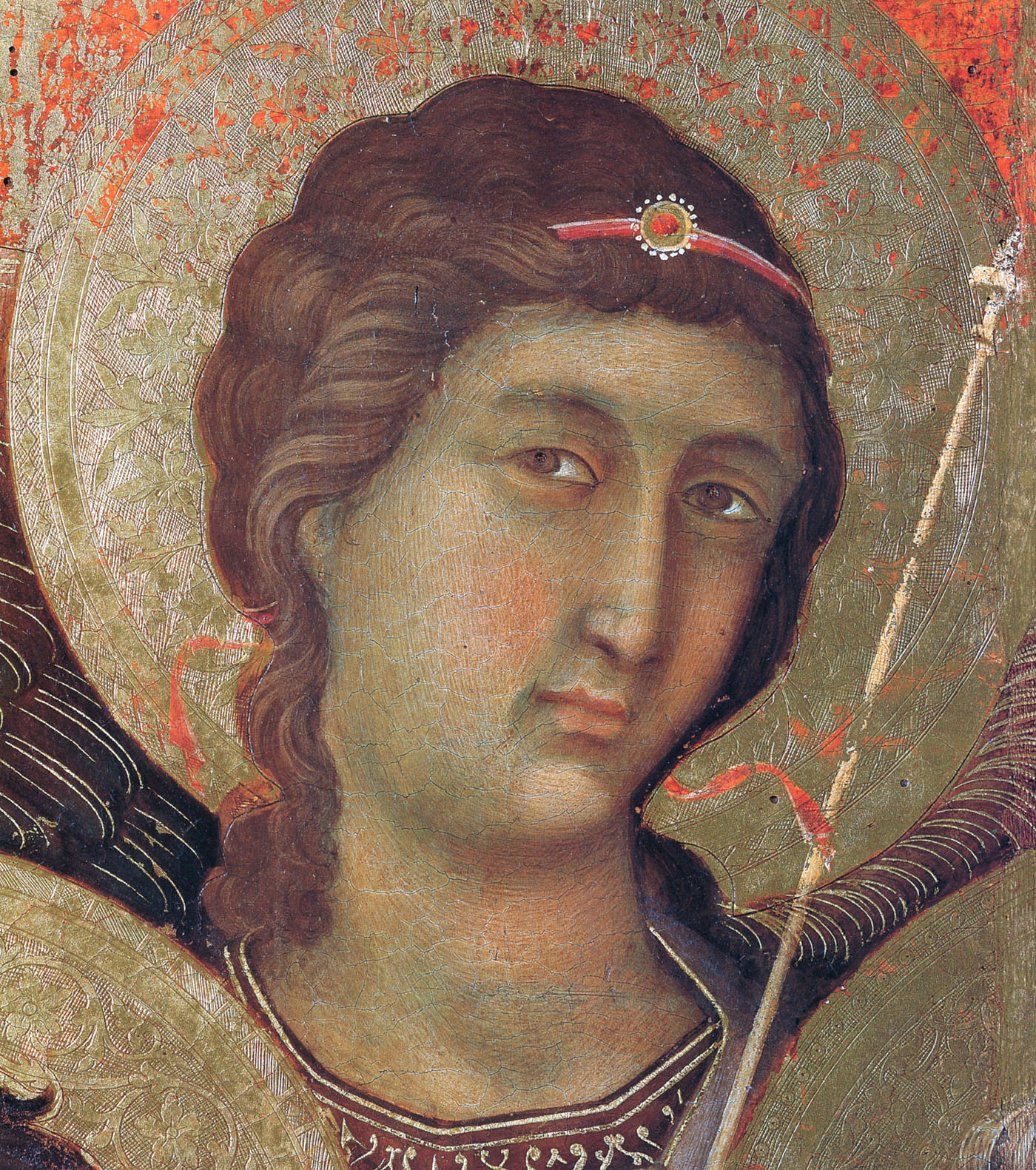This detailed oil painting by Duccio, titled "Madonna and Child on a Throne," features the close-up face of an angelic figure. Hand-painted with professional skill, the figure has light brown, wavy hair adorned with a red headband accented by a central jewel and white dots. The facial features are intriguing, blending both masculine and feminine characteristics, including light brown eyes, a longer nose, and a grayish-beige complexion.

Central to the artwork is a silver filigree halo that intricately fills the space behind the figure's head, while the background reveals red splatters and an orange hue. The face is framed by a neckline adorned with copper and silver filigree embroidery, with glimpses of ornate fabric extending to the sides.

The figure appears to hold a wand or scepter, which features a red ribbon and runs from the bottom towards the top-right corner of the image. The medium-length hair curls charmingly around the head, contrasting against a backdrop that includes colors like black, white, red, gold, pink, brown, and peach. Subtle cracks in the paint hint at the artwork’s age, likely created around 1310 during the Proto-Renaissance era. This square-format piece is both elegant and elaborately detailed, revealing Duccio’s mastery in blending figurative detail with symbolic elements.